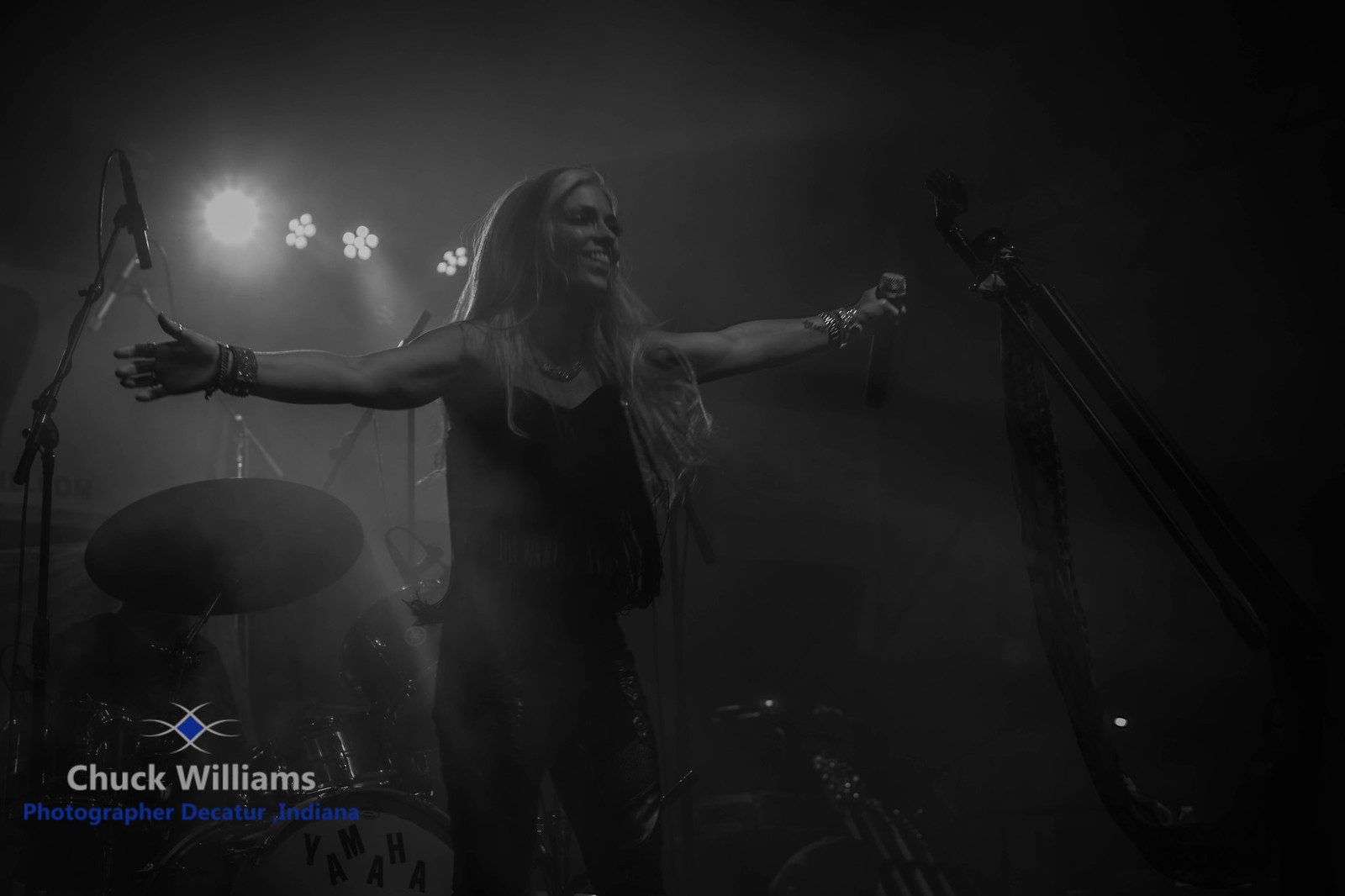This evocative black-and-white image captures a powerful rock-and-roll performance scene. The central figure is a Caucasian woman in her 30s with long blonde hair, standing slightly left of center stage, her arms outstretched as if basking in applause. She is dressed in a black tank top and dark pants, adorned with numerous bracelets, and is holding a microphone in her left hand while smiling warmly. The stage is framed by dramatic white lights behind her, casting striking rays through the darkness, creating a dynamic contrast. To her left, a drum set is partially visible, including a cymbal and branding like 'Yamaha.' A microphone stand with a draped scarf stands before her, adding to the rock-and-roll ambiance. In the bottom left corner, the logo reads, “Chuck Williams, Photographer, Decatur, Indiana,” anchoring the image's authenticity. The lighting details and stage equipment hint at a vibrant musical performance, with the woman's poised stance suggesting she has just finished an electrifying song.